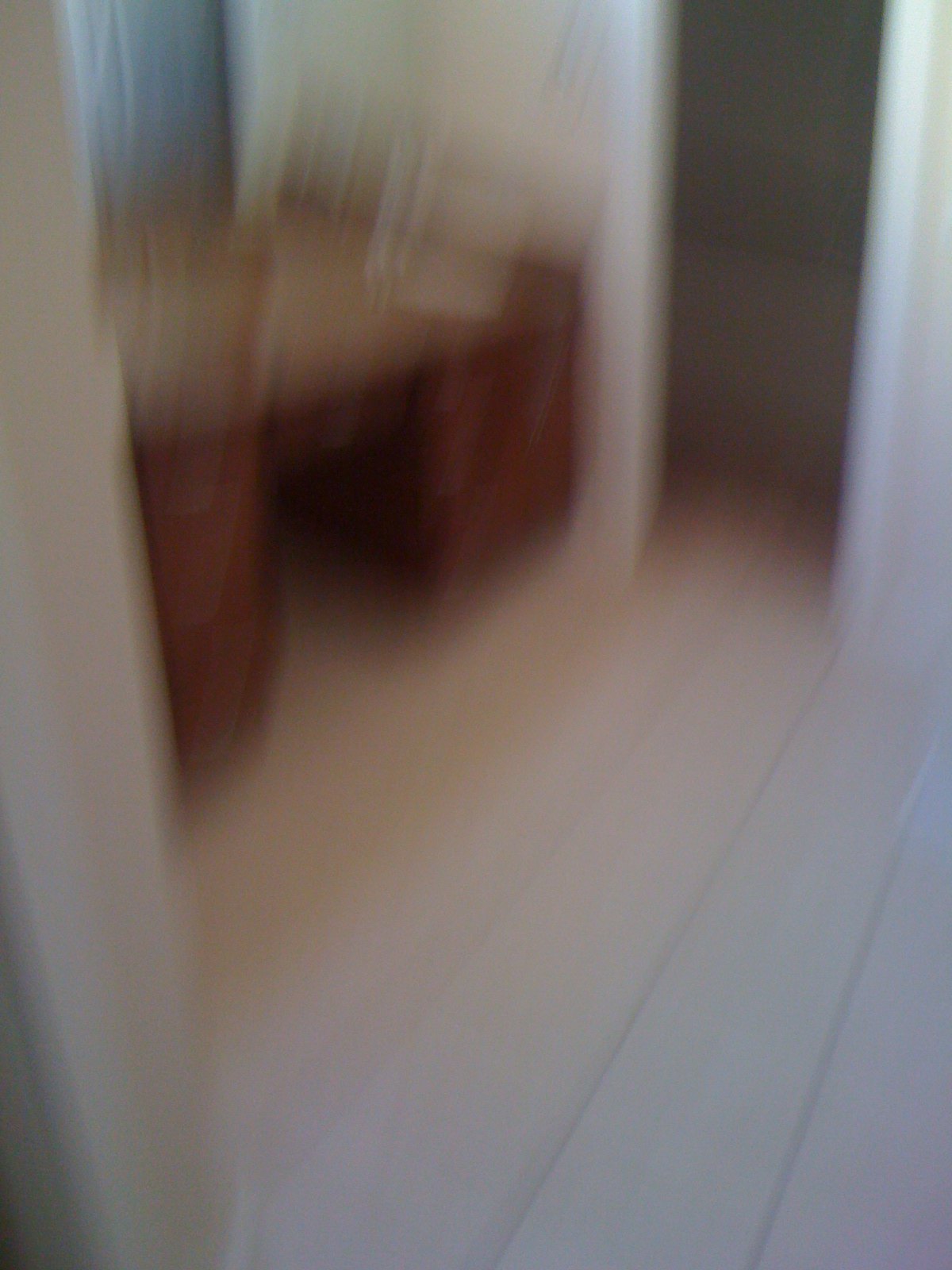In the image, despite its notable blurriness, a small, somewhat clear room is visible. The floor is a lighter colored wood. Dominating the space is a wooden desk, which might also be a vanity, centrally positioned against the wall. The desk features a single drawer in the center, with additional drawers organized in pairs on either side. Behind this furniture piece hangs a blue curtain, which may appear gray due to the image's quality, providing a wispy, thin window treatment. The walls of the room are a light beige or cream color, adorned with white trim. On the left side of the room, there is a doorway trimmed in white, leading to another small space which might be a closet or another room. This secondary area shows a hint of something white, potentially resembling a bathtub, juxtaposed with an ivory-colored towel on the floor, suggestive of a bathroom.